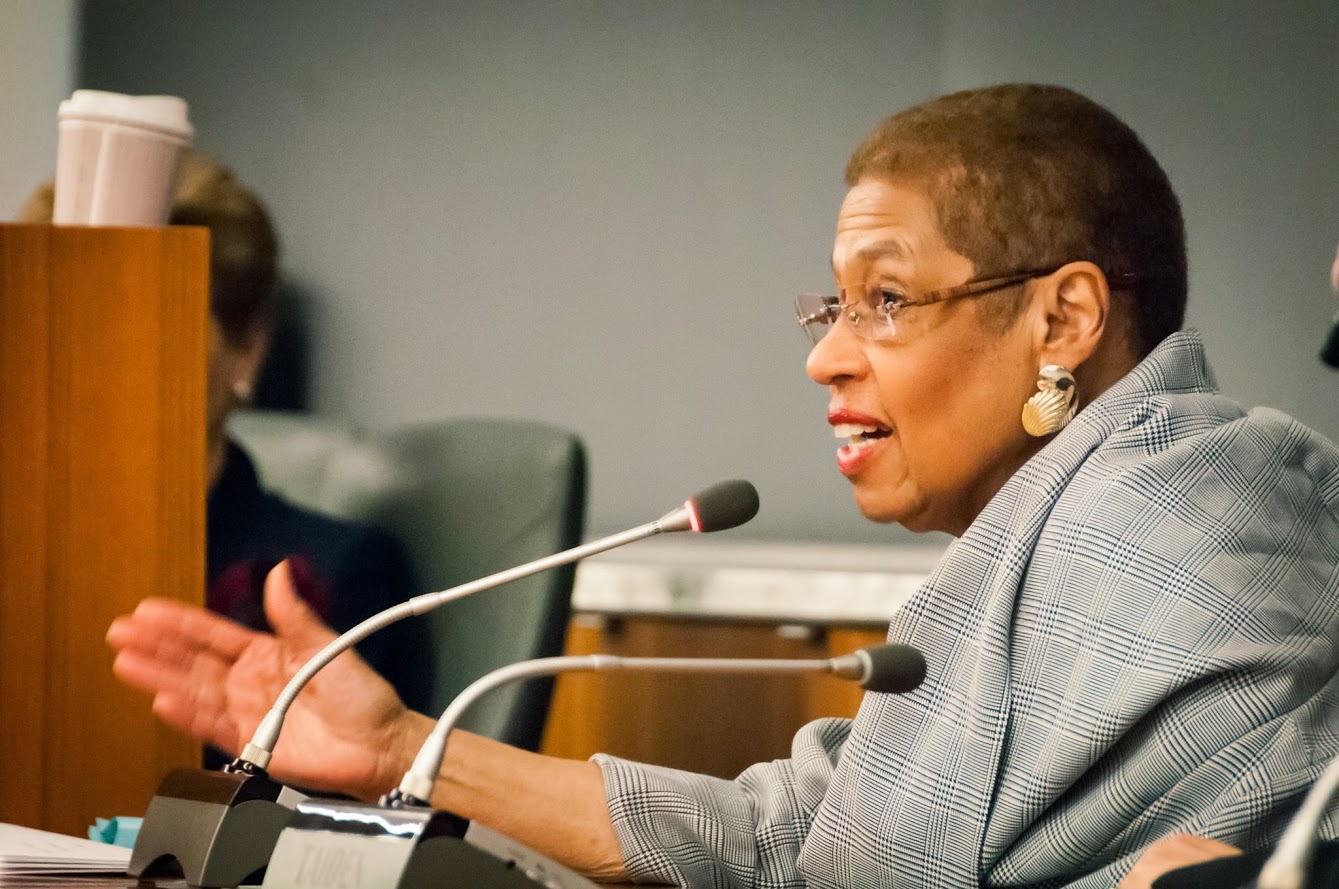The photograph captures an African-American woman speaking passionately into a microphone at what appears to be an indoor setting, possibly a courtroom or council meeting. The woman, slightly dark-skinned with very short, cropped hair, occupies the right half of the image. She's wearing glasses with dark frames, bold red lipstick, and large gold earrings shaped like seashells. Draped over her shoulders is a gray and dark blue plaid shawl. The woman’s right hand is raised with her palm up, emphasizing her animated speaking. In front of her are two adjustable stand microphones, with one directed towards her and the other aimed at an individual partially visible by a hand, cut off by the image's edge. To her left, partially obscured by a divider, sits another person on a green chair and a black chair is seen further left, next to a podium with a styrofoam cup that likely contains a drink. The background hints at a formal setting, marked by the presence of wooden desks suggestive of a courtroom environment.